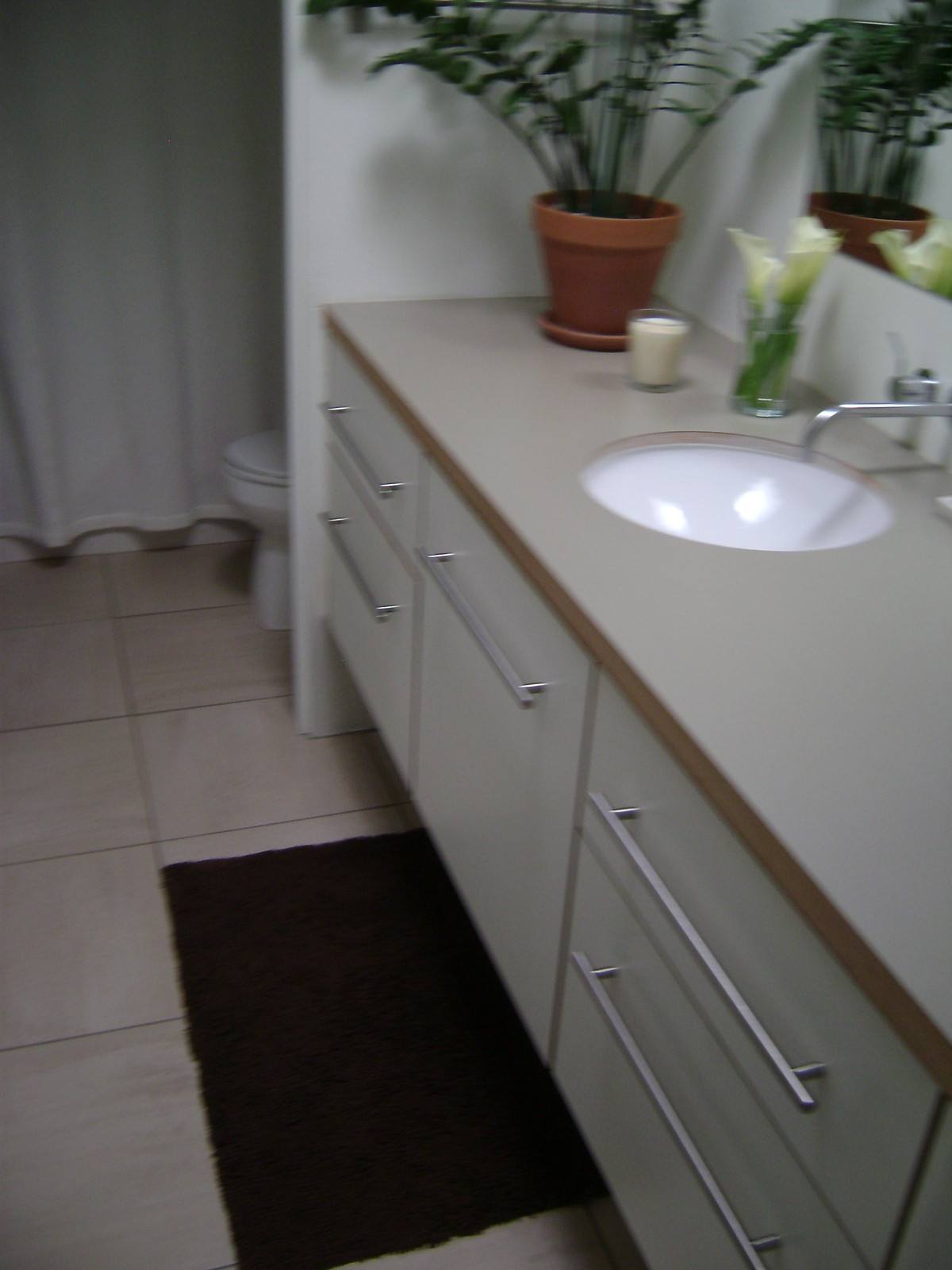The image showcases a meticulously clean and contemporary bathroom. The space features cream-colored cabinetry adorned with large, modern silver pulls, contributing to a sleek aesthetic. The bathroom boasts a sunken sink paired with an elegant, modern faucet and handles. A sizable potted plant occupies a corner, casting a soft shadow on the pristine white walls that harmonize with the white shower curtain and sink. 

Adding a touch of nature, a glass vase filled with water holds fresh flowers, while a cream-colored candle enhances the ambiance. The reflection of the plant in the mirror further amplifies the room's serene atmosphere. The flooring consists of large, high-quality tiles, partially covered by a brown throw rug positioned in front of the sink. The white toilet is visible in the background, completing the scene of this clean and stylish bathroom. The countertop on the right remains uncluttered, emphasizing the room's neat and orderly appearance.